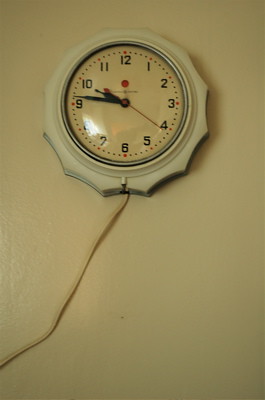This photograph showcases a uniquely designed clock hanging on a wall. The clock features a white exterior with a distinctive shape, resembling a stylized sun with circular cutouts around its perimeter. A cord dangles down from the clock's center. The clock face, protected by a glass cover, is an off-white or ecru color. It displays Arabic numerals from 12 to 11, with small dots connecting each numeral around the circumference. The current time shown on the clock is approximately 10:45 or 10:46. Additionally, red dots are positioned at each hourly marker. The clock also includes a second-hand dial, adding to its functionality and intricate design.